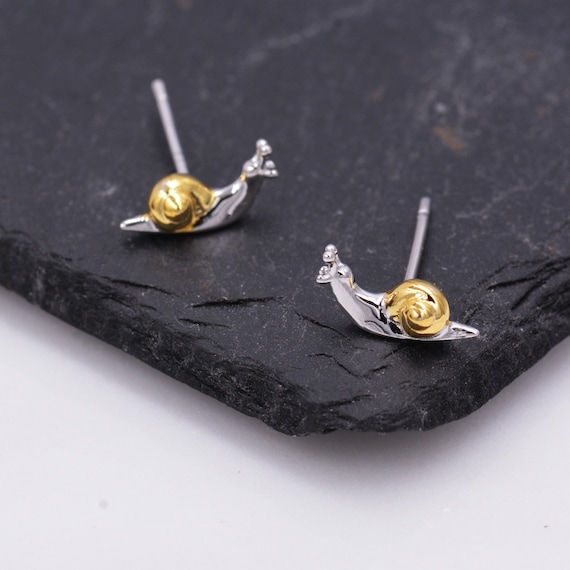This image showcases a pair of small, meticulously crafted, snail-shaped metal items that could be either earrings or cufflinks. Each snail features a shiny silver body and a golden shell, with a long silver post extending from their backs. Positioned on a textured black slate or rock with deep crevices and a natural grainy appearance, they stand out strikingly against the stark white background. The snails face opposite directions and cast subtle shadows on the black surface. With their polished, contemporary design, these pieces are ideal for shopping platforms like Etsy, intended to capture the eye with their unique blend of elegance and whimsy.